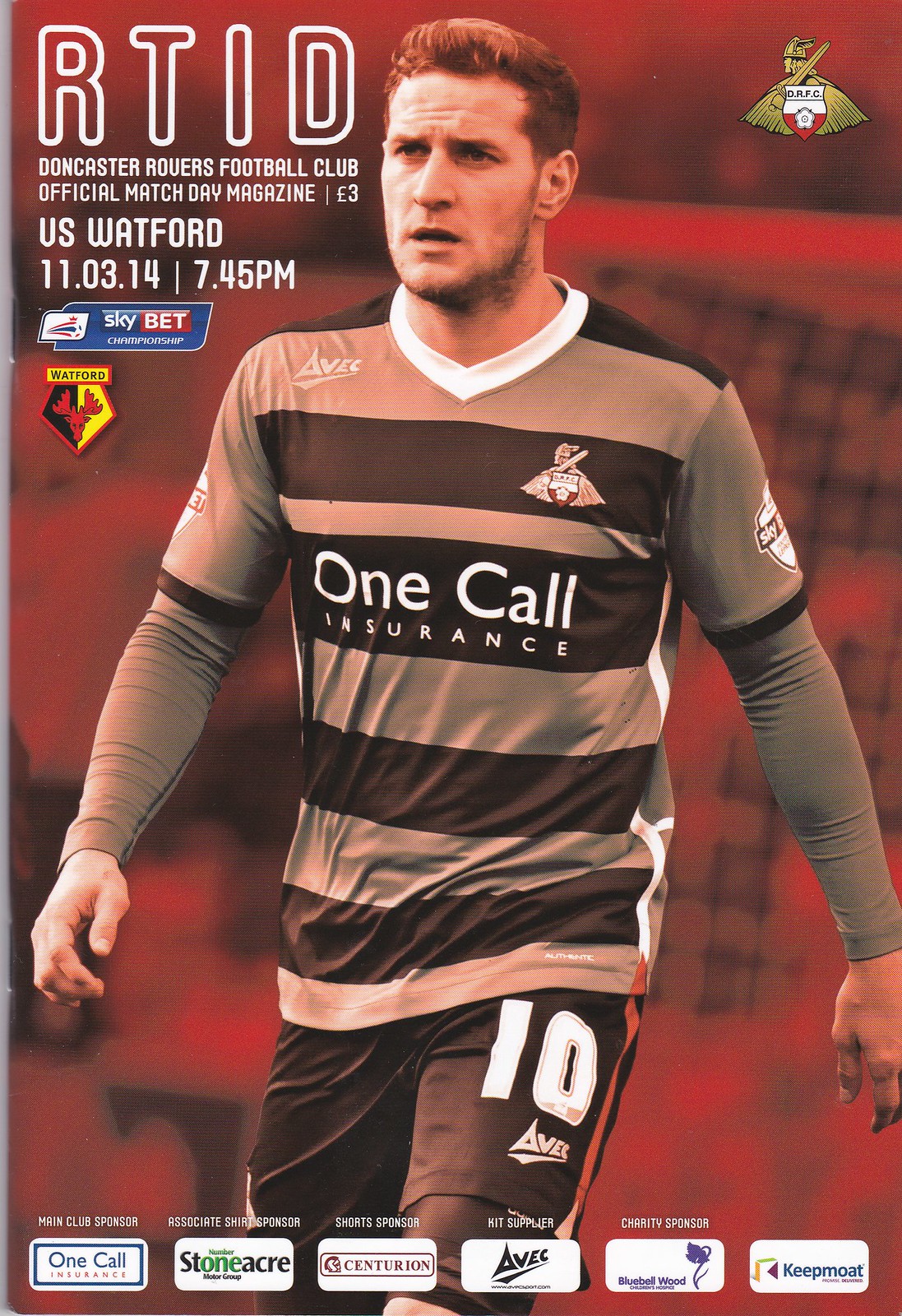This vertically-aligned rectangular image serves as the cover for a Doncaster Rovers Football Club match day magazine, predominantly featuring a muted red background. At the center of the cover is a full-page photograph of a soccer player with reddish hair, clad in brown shorts and a striped brown and dark brown shirt. Emblazoned on his shirt in white lettering is the team sponsor "One Call Insurance." 

The top left corner of the magazine displays the title "RTID" in bubble letters with a red background outlined in white. Below this, in smaller white text, it reads "Doncaster Rovers Football Club Official Match Day Magazine" followed by the details "Versus Watford - 11.03.14 - 7:45 PM." The top right corner features an insignia with a diamond-shaped logo displaying deer horns, half in black and half in yellow, outlined in red with "Watford" above it. Beneath this, a small blue logo for "Sky Bet" appears, though the words under it are unclear.

The sponsors listed at the bottom of the cover include "One Call Insurance," "Stone Acre," "Centurion," "AVEC," "Blue Ball Wood," and "Keepmote." Further down, the player's shorts also display the sponsor "AVIA" along with the number 10 in white. The overall red-tinted background features subtle elements, potentially a checked pattern or netting, that add to the visual complexity without allowing any single element to dominate.